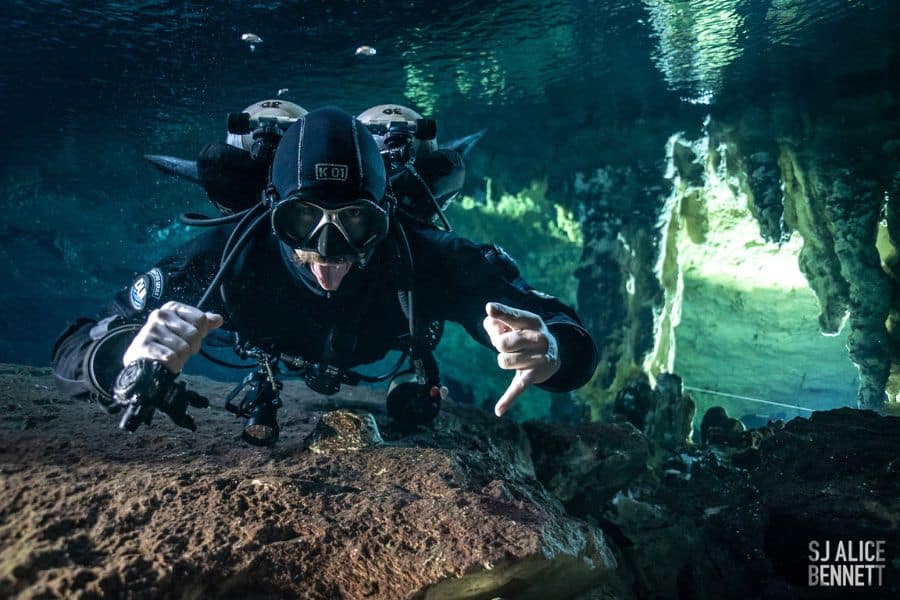The image captures an underwater cave scene where a man in full black scuba diving gear poses mid-dive. The diver is floating horizontally, facing the camera with his tongue out and his right hand forming the rock star hand symbol, while his left hand holds his breathing apparatus. His black goggles and oxygen tanks are clearly visible. The eerie, dark underwater cave surrounds him, with light filtering in from the right and stalactites hanging from the ceiling. Rocks and corals line the ocean floor beneath him, and a couple of air bubbles are seen rising upward. "S.J. Alice Bennett" is inscribed in the bottom right corner of the photograph.